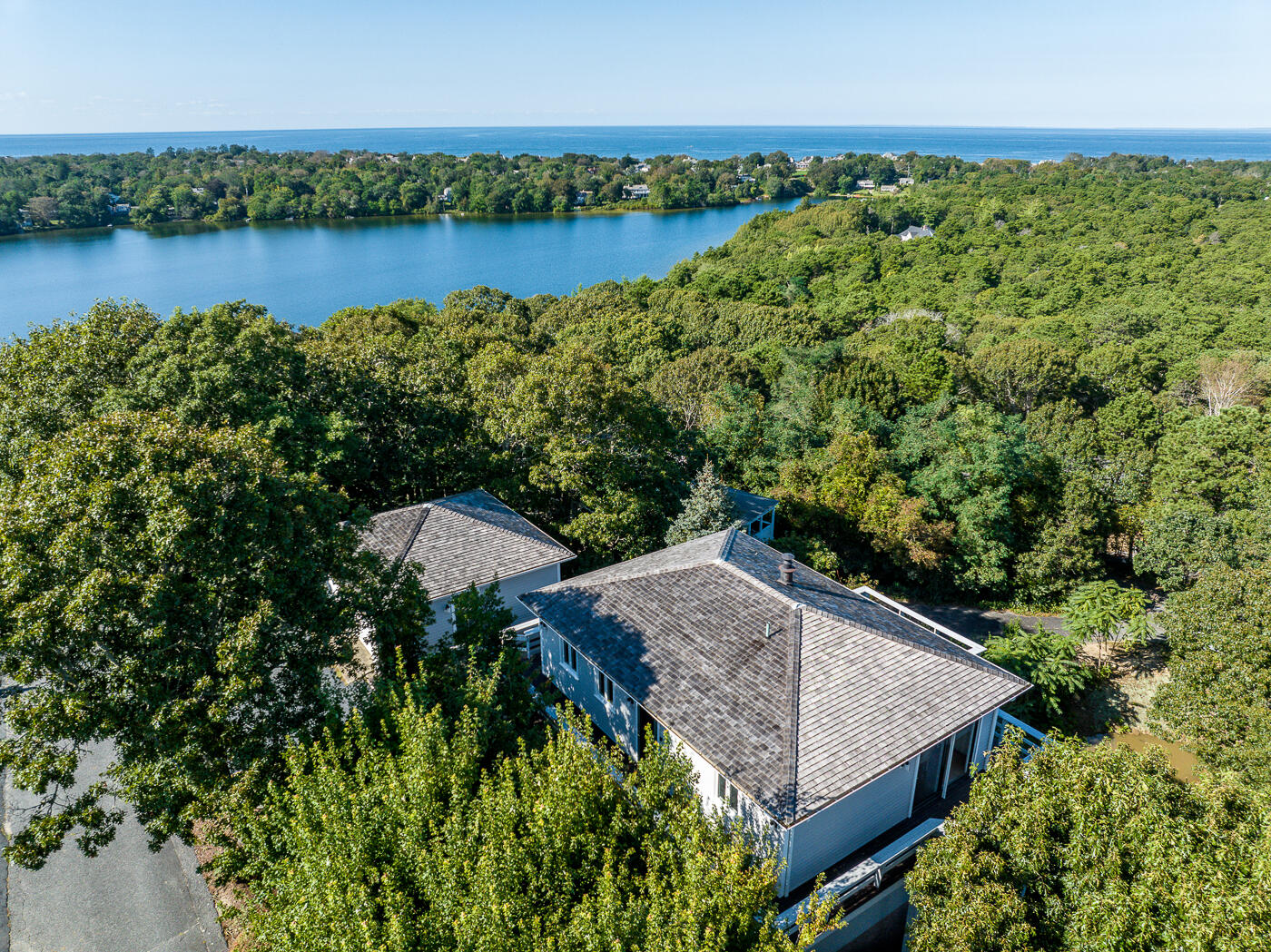The aerial photograph captures a striking view of a large, multi-storied house with white walls and a gray roof, nestled in the heart of a lush, vibrant green forest. Beside this main house is a smaller single-story building, which resembles a barn. The scene is framed by a vast expanse of healthy, thriving trees, creating a serene and secluded atmosphere. The landscape is dotted with large bodies of clean, dark blue water, possibly part of a delta system, that extend towards the horizon where they meet a clear, light blue sky. To the upper left, the water appears to open into what might be the open sea, while in the lower right, the edge of a road hints at civilization. In the distant background, a few more houses can be glimpsed across the water. The overall scene is one of natural beauty and tranquil isolation.